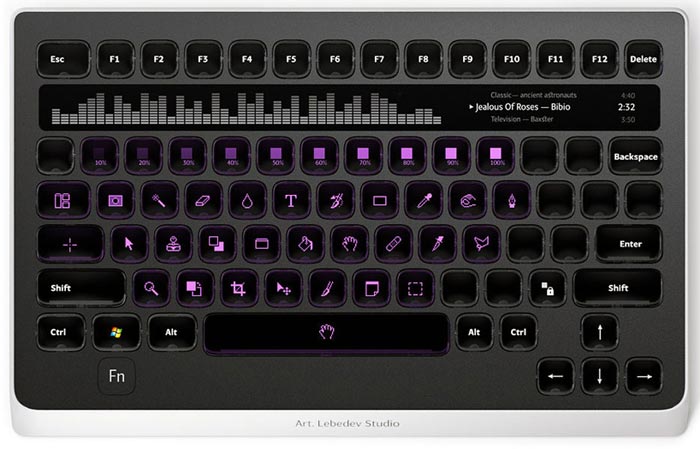The image depicts a unique, dark-hued keyboard with black buttons featuring white or pink labels. The top row consists of function keys labeled F1 through F12, starting with the Escape key on the far left and ending with the Delete key on the far right. Directly below this row is a small screen displaying a bar graph and the currently playing audio track titled "Jealous of Roses" by Bibio, with a duration of 2 minutes and 52 seconds. 

The keys beneath this screen are primarily decorated with pink symbols rather than traditional letters or numbers. The right-most key in this row is designated as the Backspace key. The row below continues with more pink symbols, though the three keys on the far right are blank. The fourth row includes an Enter key on the far right and blank keys just to the left of it, interspersed with keys bearing pink symbols. 

The penultimate row starts with a Shift key on the far left, followed by a series of keys with pink labels, transitioning to two blank black keys, and culminating with another Shift key on the far right. The bottom row features the Control key on the far left, followed by the Windows key, the Alt key, a space bar marked with a pink hand symbol, another Alt key, and another Control key. In the lower right corner, the traditional arrow keys are present, while the bottom left corner houses an Fn key. The design hints at a specialized use, like a mixing keyboard for a musical artist or a unique computer interface created by Art Lebedev Studio.